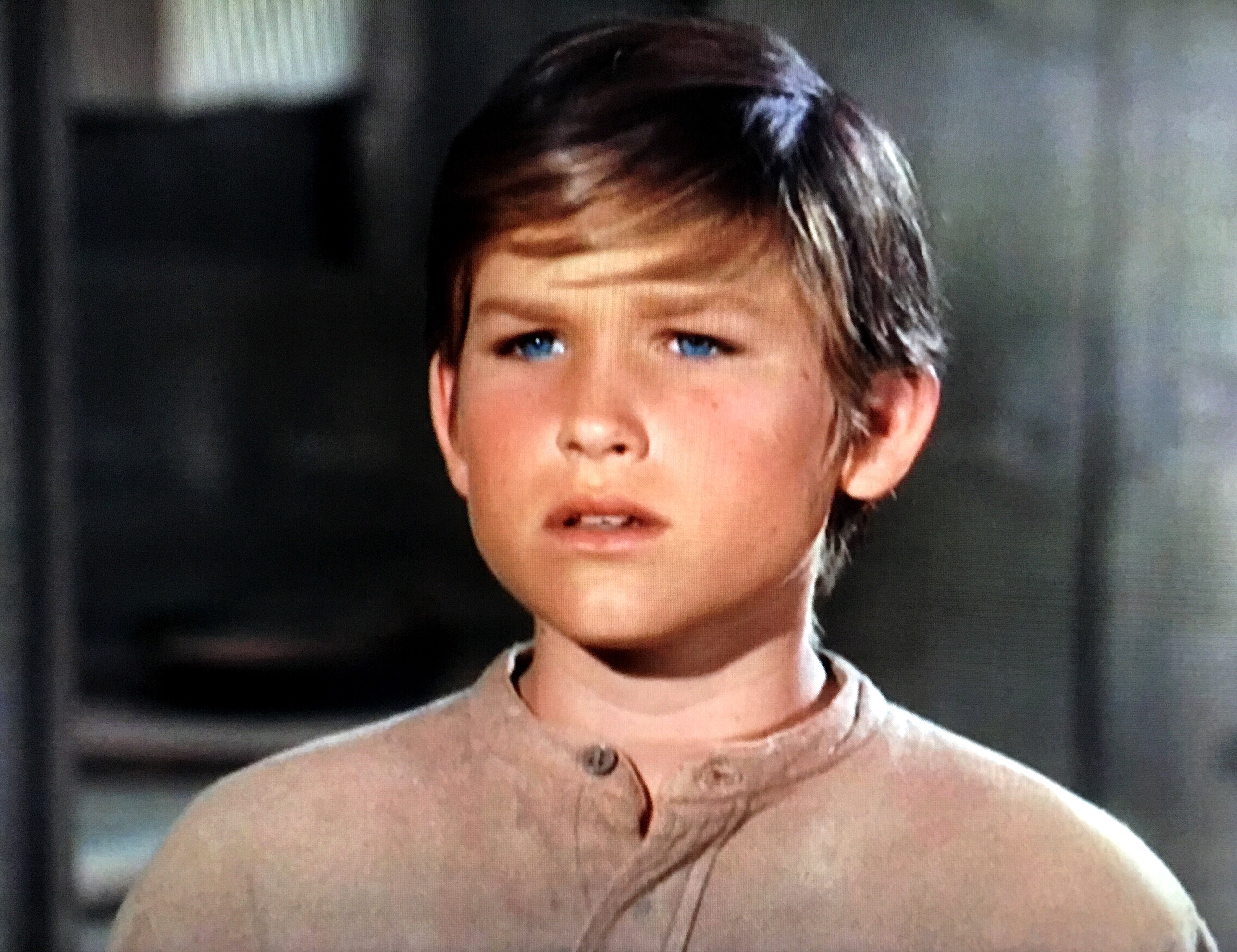This photographic image, possibly a still from a movie or TV show, captures a young white boy who bears a resemblance to a young Kurt Russell. He appears to be around 9 or 10 years old and has striking blue eyes, short dirty blonde hair, and an expression that conveys sadness. The boy is standing indoors, slightly oriented away from the camera. He wears a brown shirt with a gray button and a collar, which is partially unbuttoned, revealing a white undershirt beneath. His mouth is open, showing two of his teeth. The background features gray wooden planks and what could be a window, suggesting a rustic, homey room setting.